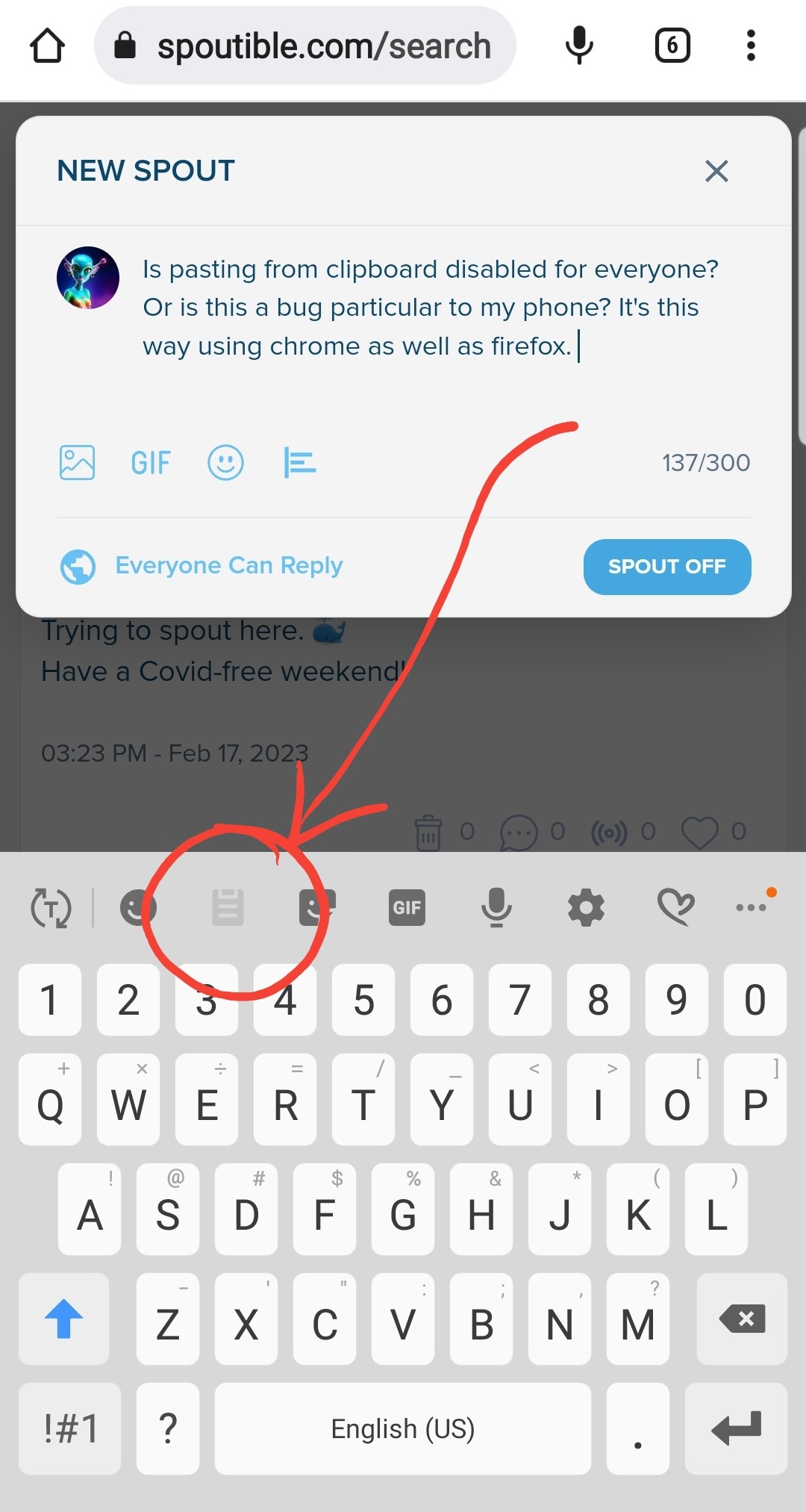A detailed screenshot from a cell phone captures the user interface of the Spoutible website. At the top of the screen, a house icon is visible next to a search bar containing a black padlock on the left side and the URL "spoutible.com/search" inside it. On the right side of the search bar, there are three elements: a microphone icon, a black square with the number "6" inside, and a vertical trio of black dots.

A prominent white pop-up window titled "New Spout" is centered on the screen. The text within it questions, "Is pasting from clipboard disabled for everyone, or is this a bug particular to my phone? It's this way using Chrome as well as Firefox." The pop-up shows a character count of "137/300," indicating the number of characters used out of the allowed 300. Below this is the label "Everyone can reply," and at the bottom of the pop-up, there's a blue rectangle with the text "Spout off" in white letters.

A red arrow, drawn by someone, points downward towards the toolbar just above the phone's keyboard. The red arrow highlights a red circle that encases a grayed-out clipboard icon. This part of the screen shows that the clipboard functionality is disabled. 

The pop-up obscures a partial conversation in the background, which reads, "Trying to spout here" followed by an emoji of a whale. Another visible message wishes, "Have a COVID-free weekend," dated "February 17, 2023," at "3:23 PM."

At the very bottom of the screenshot is the phone’s keyboard, indicating that the user was in the process of typing.